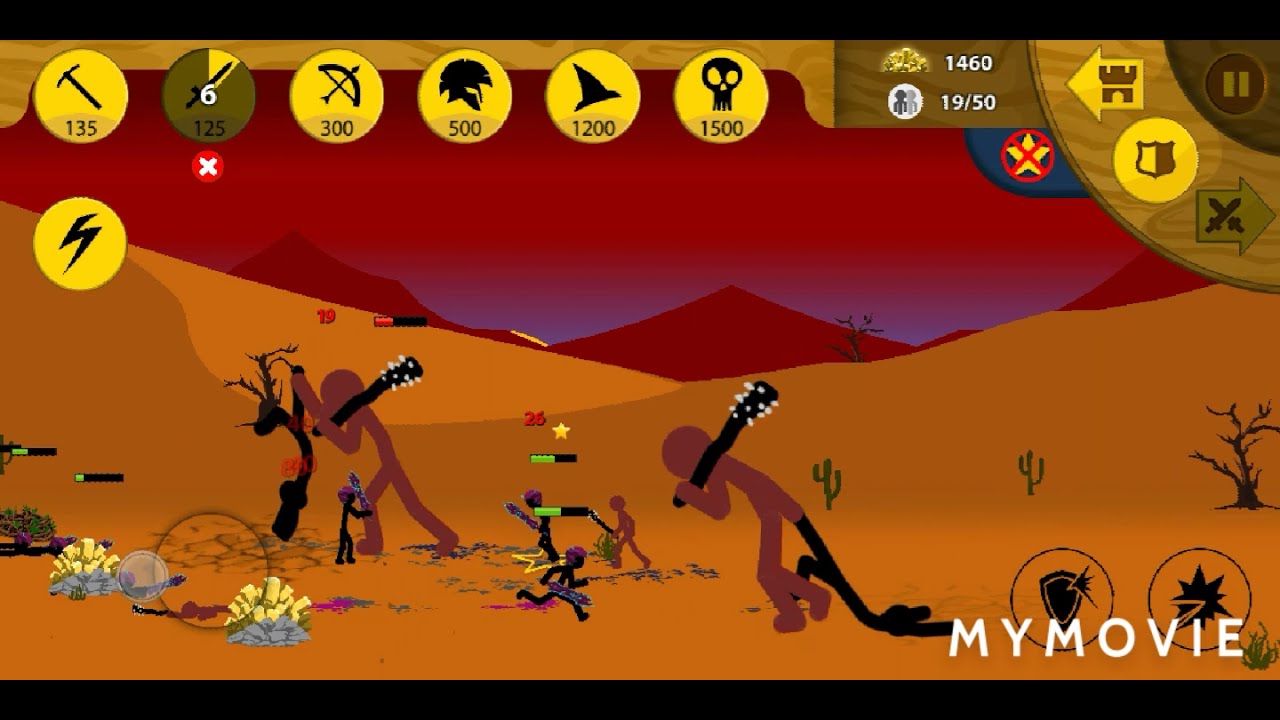This image is a detailed screenshot from a video game, specifically an app game, set in a dark yellow desert area reminiscent of a classic jazz album cover with a Picasso-like aesthetic. The scene is filled with stick figure characters, depicted with simple line bodies, circular heads, and two limbs each. The characters are either tall and purple or short and black, engaged in combat. The taller figures wield crude spiked clubs and drag the shorter ones, who hold small knives and charge at their larger adversaries. Each small figure has a health bar above its head.

The desert landscape is sparsely populated with cactus plants and dry trees, and the sky is red with distant, red-tinged mountains in the background. Various icons adorn the top of the screenshot, including symbols like a bow and arrow, a Roman helmet, a witch's hat, a skull, and a pickaxe, each paired with numbers indicating scores or quantities (e.g., pickaxe 135, arrow 300). To the right, there is a score display that reads "1460" and a ratio "19/50". The watermark "MY MOVIE" is prominently placed in white text in the bottom right corner.